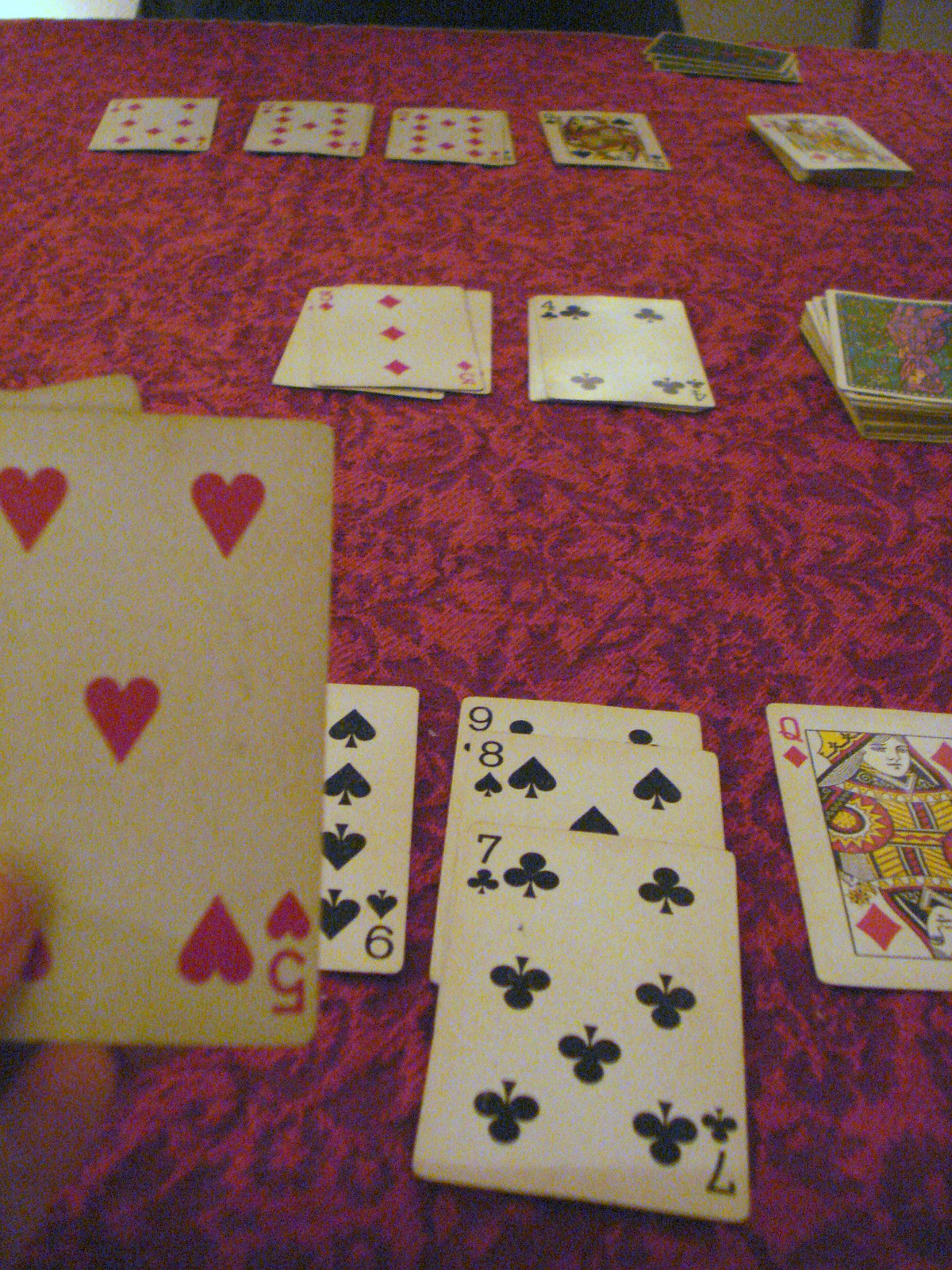The image depicts a game of Solitaire displayed on a table with a purple, velvet-like covering adorned with floral patterns. The layout of cards follows the traditional Solitaire format. In the upper portion of the scene, a deck of cards is partially visible. On the tableau, there is a Queen of Spades adjacent to a Nine of Diamonds, followed by what appear to be an Eight and Seven of Diamonds, though the latter cards are somewhat blurred.

Central to the image are a Three of Diamonds with a few cards below it, and a Four of Clubs next to a larger deck of face-down cards. In the foreground, a hand, likely belonging to the unseen player, holds a Five of Hearts. The spread of cards in the player's hand includes a Nine of Clubs, Eight of Spades, Seven of Clubs, Nine of Spades, and a Queen of Diamonds. The overall setting and clarity of the card game suggest that this is indeed a game of Solitaire, though it is ambiguous whether there is a second player involved given the positioning and arrangement of the cards.